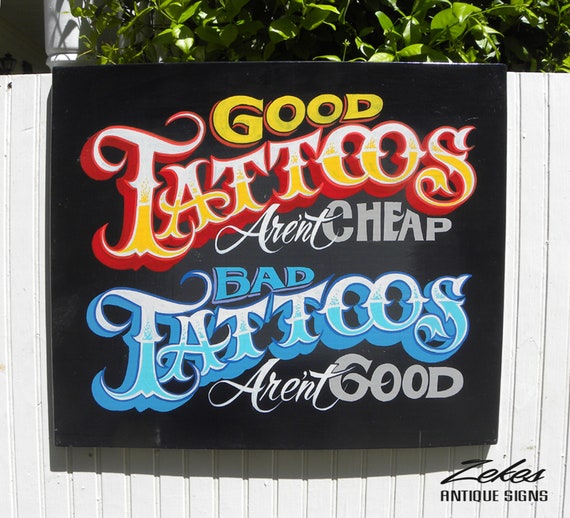A black sign with ornate lettering hangs on a white painted fence, partially obscured by green foliage visible above and behind the fence. The sign's message reads, "Good Tattoos Aren't Cheap, Bad Tattoos Aren't Good." The words "Good" and "Tattoos" are prominently featured in vibrant, stylized fonts, with "Good" in yellow outlined in red and "Tattoos" transitioning from white to yellow and outlined in red. "Bad Tattoos" appears in blue, outlined by white, with "Bad" in a darker blue and "Tattoos" transitioning from white to a lighter blue. A small text at the bottom right of the sign credits "Zeke's Antique Signs." A white pillar stands to the left of the sign, contributing to the image's overall aesthetic.